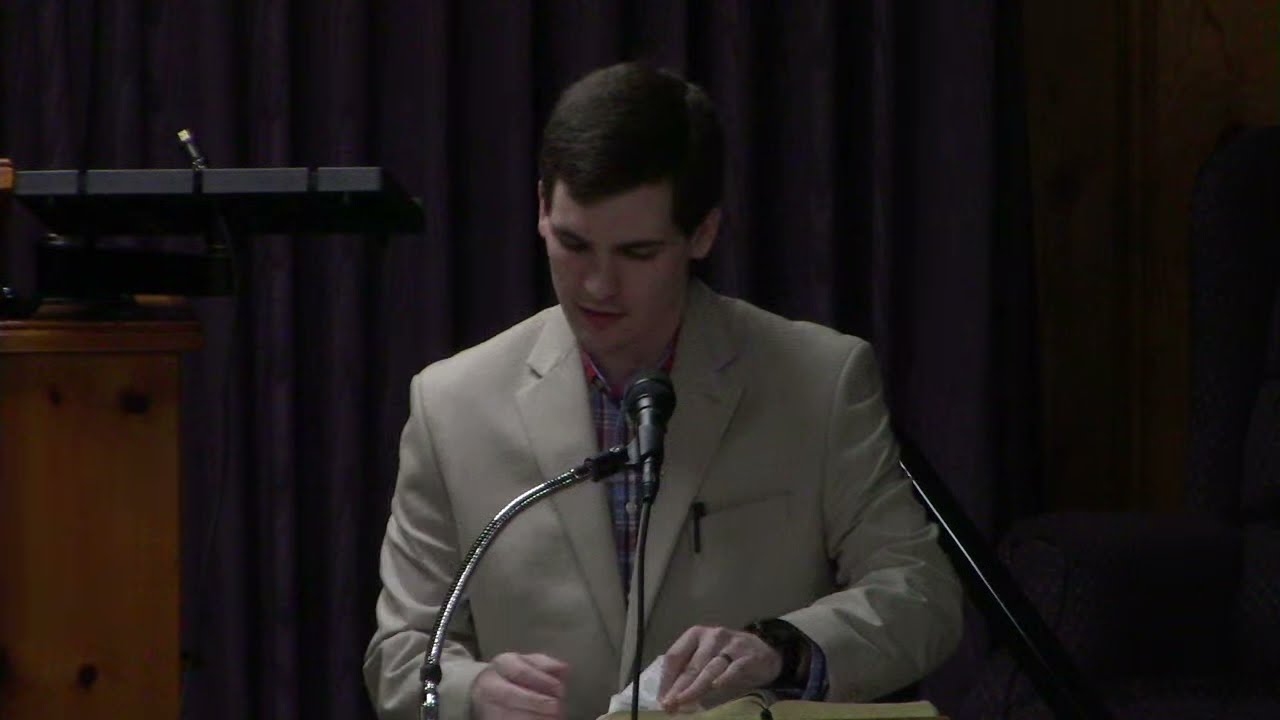The photograph depicts a young, light-skinned man in his late 20s to early 30s, standing at a podium and seemingly giving a speech. He has short, dark hair with a widow's peak and is dressed in a beige or whitish-gray suit jacket over a button-down plaid shirt. Notably, the man is wearing a wedding ring on his left hand and has a pen tucked into the chest pocket of his blazer. He is looking down, appearing to read from a book, possibly a Bible, while addressing the audience through a black microphone with a curved base. The setting includes a dark backdrop with black curtains and a keyboard placed atop a tall wooden pedestal behind him, adding to the formal atmosphere. The image is a color photograph in landscape orientation, capturing a moment of thoughtful oration with a focus on the subject's detailed attire and surroundings.